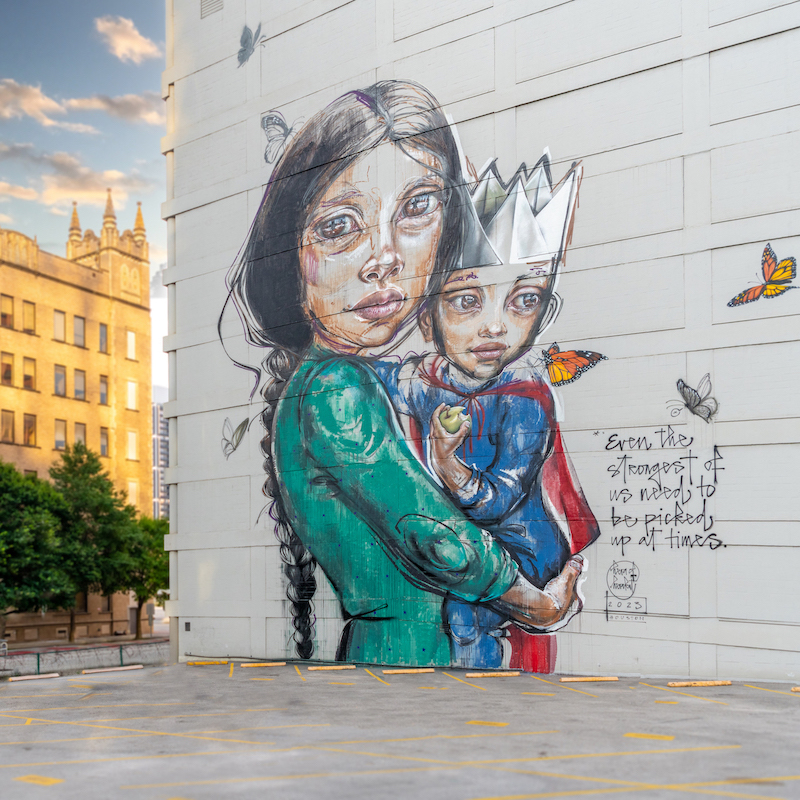The photograph showcases a vibrant mural on the white, square-patterned exterior wall of a building. The mural illustrates a heartwarming scene of a Hispanic woman with dark, long hair styled in a pigtail braid, dressed in a long-sleeved green dress. She lovingly holds a young Hispanic boy, roughly three or four years old, who is adorned in blue pajamas, a bright red cape, red boots, and a silver crown. The boy also clutches an apple in one hand. To their right, a cluster of monarch butterflies flutters, complementing the touching message written in cursive: "even the strongest of us need to be picked up at times," dated 2023. Across the street to the left, a multi-story, gold-colored building with a cathedral-like top punctuates the urban landscape. Above, in the left corner of the photo, patches of clouds drift through the sky.